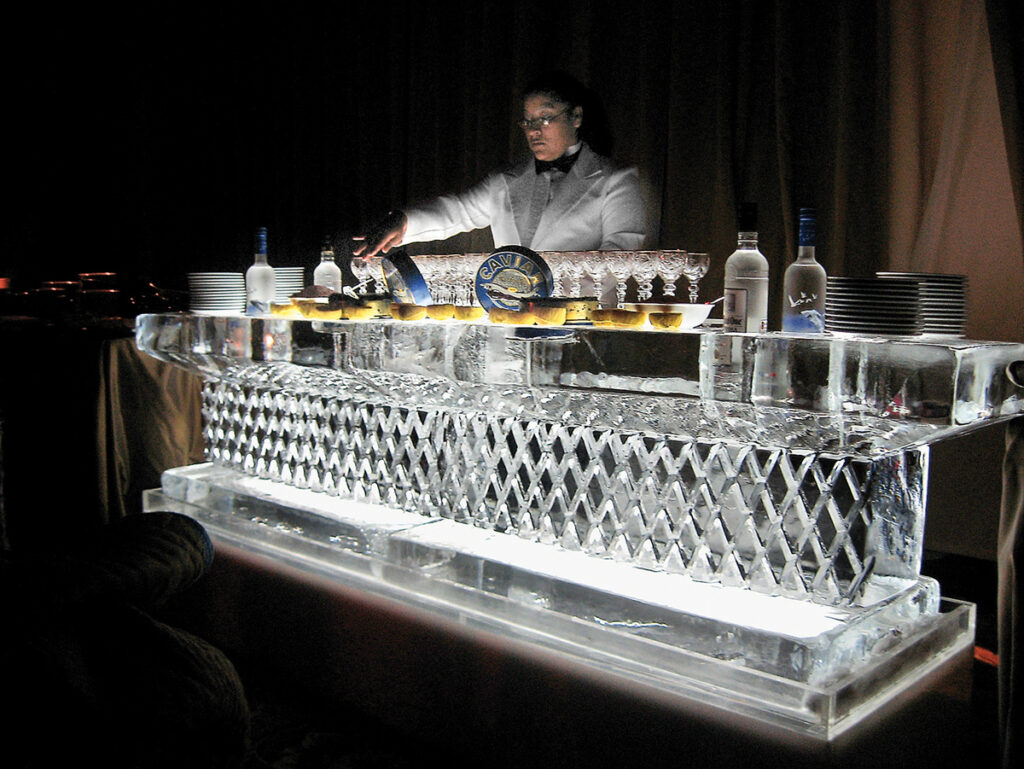In a dimly lit room, an intricately sculpted ice bar gleams under strategic lighting, creating an ethereal ambiance. Taking center stage at the luminous bar is a bartender, donned in a white jacket reminiscent of a tuxedo, complete with a black bow tie. His dark hair is neatly groomed, and he wears small circular glasses perched slightly down his nose. The bartender's right arm extends forward, his hand delicately touching a glass on the bar's surface, which is dotted with an array of wine glasses and a few bottles of clear liquor. The bar itself, gleaming like crystal, features a lattice design, enhancing its glass-like appearance. Positioned behind the bartender is a brown curtain that accentuates the dark surroundings, while the light beneath the bar creates a striking visual contrast, making the ice structure appear almost surreal.